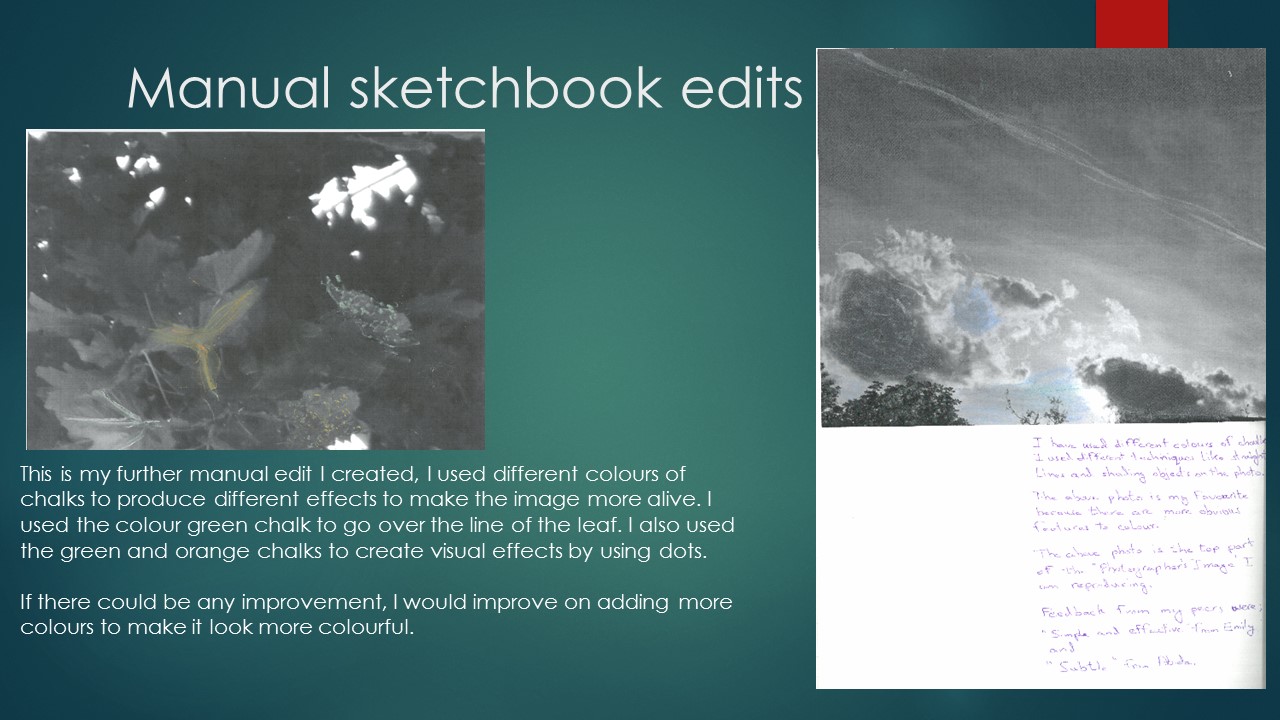The PowerPoint slide features a detailed template background composed of a blue color with a green circle in the center and a red banner positioned at the top right. At the top, written in white text, the heading reads "Manual Sketchbook Edits." 

On the left side of the slide, there is a square, scanned image that depicts leaves, a tree, and light filtering through the gaps in the foliage. Below this image is a white paragraph stating, "This is my further manual edit I created. I used different colors of chalks to produce different effects to make the image more alive. I used the green colored chalk to go over the line of the leaf. I also used the green and orange chalks to create visual effects by using dots." The text follows with a separated sentence: "If there could be any improvement, I would improve on adding more colors to make it look more colorful."

On the right side of the slide, there's an A4 sheet image with sky imagery at the top, showing clouds and light with some marks and lines, as well as the tops of trees in the corner. The bottom half of the page contains unreadable text written in blue pen. These details are accompanied by a few paragraphs on the right side.